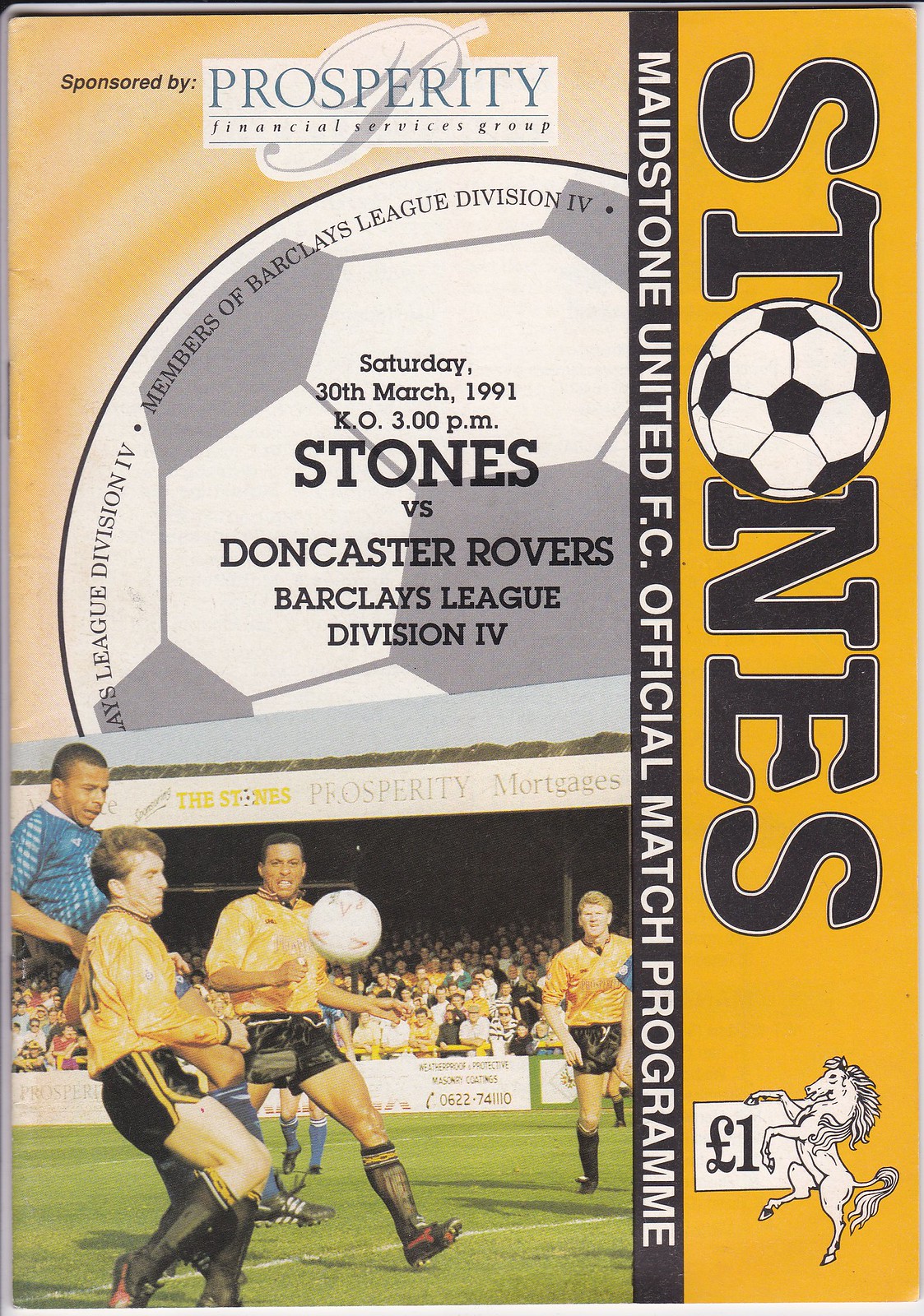The image depicts the front page of a soccer match program. The top section has a yellow background, prominently displaying the text "Prosperity Financial Services Group" as the sponsor. To the top right, there's an image of a gray and white soccer ball, encircled by the text "League Division IV, Members of Barclays League Division IV." In the center of the soccer ball, detailed information about the match is provided: "Saturday, 30th March 1991, K.O. 3 p.m., Stones versus Doncaster Rovers, Barclays League Division IV."

On the bottom left-hand corner, there is a color image of a soccer match in progress, showing around four or five players on green grass, dressed in yellow shirts, black shorts, black socks, and black shoes. A black vertical bar on the right-hand side of the image features the text "Maidstone United FC Official Match Program" in white letters. The word "Stones" is written vertically, with the letter 'O' replaced by a soccer ball. In the bottom right-hand corner, an image of a horse holding a sign that reads "1 Pound" is visible.